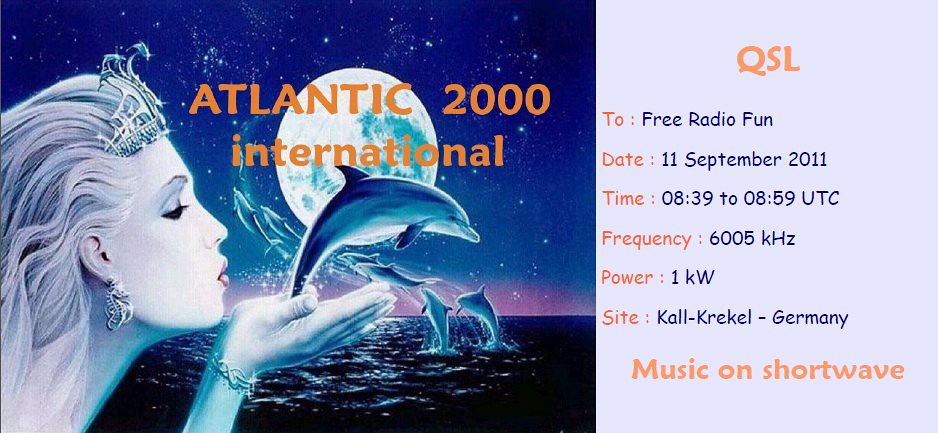The advertisement features an enchanting night scene with a stylized image of a woman on the left, blowing a kiss, from which a dolphin emerges. The background reveals an ocean bathed in moonlight under a night sky adorned with a full moon. Several dolphins can be seen leaping out of the water, heading towards the moon. The horizon glows faintly with a hint of purple, suggesting the sun has just recently set. 

To the right of the image, a section of light purple or lavender hosts the event details in a mix of orange and blue text. At the top, "Atlantic 2000 International" is prominently displayed in orange. Beneath that, "QSL 2" appears in orange text, followed by "Free Radio Fun" in blue or blackish text. Further below, details about the broadcast are given:
- **Date:** 11 September 2011 (in blue text)
- **Time:** 0839 to 0859 UTC (in blue text)
- **Frequency:** 6005 kHz (in blue text)
- **Power:** 1 kW (in blue text)
- **Site:** Kahl Krekel, Germany (in blue text)

At the bottom, a final note in orange text reads, "Music on shortwave." The overall design merges whimsical art with essential broadcasting information, creating an intriguing and visually appealing advertisement.